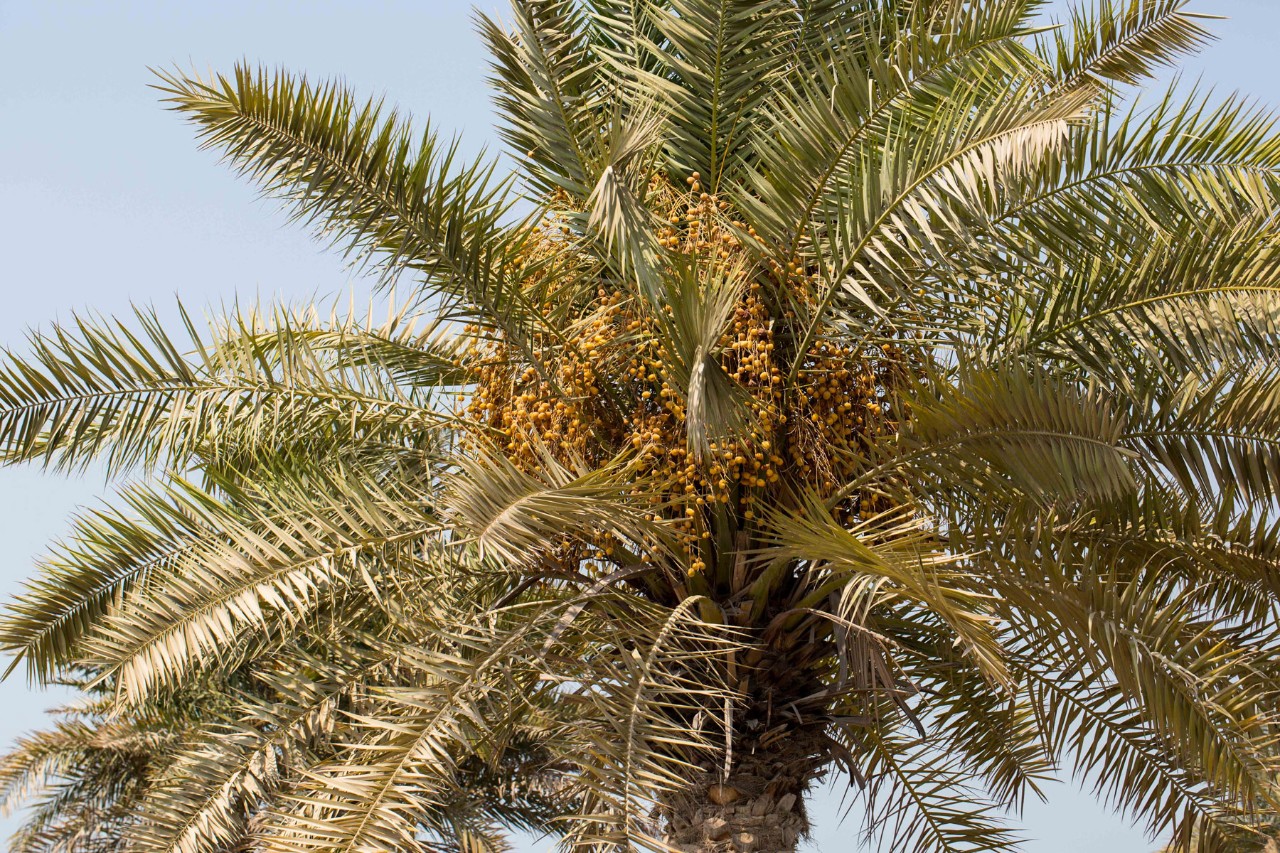This color photograph captures the top part of a palm tree, with only a small portion of the trunk visible at the bottom center. The majority of the image is dominated by numerous palm branches extending out in every direction from the tree's center. These branches are long and thin with sharp, bladed leaves. Amongst the branches, clustered towards the center of the tree, are hundreds of small, orange balls, likely fruits or seed pods. The arrangement of the leaves varies, with some branches curving downward and others projecting upward, particularly noticeable with some barren spots on the top left side. The background features a light blue sky, providing a serene backdrop to the intricate details of the palm tree's foliage and fruit.